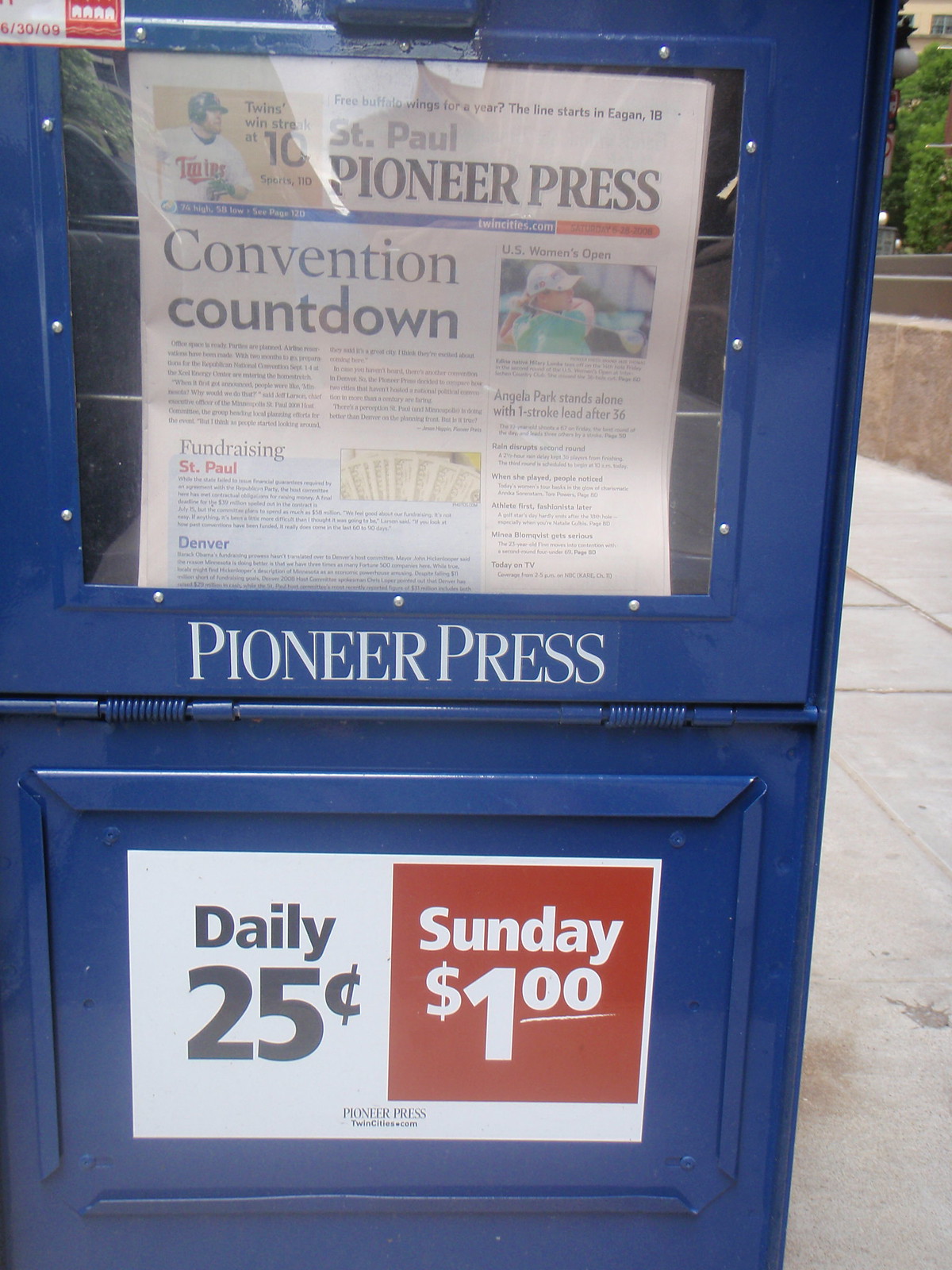This detailed photograph captures a blue, metal newspaper dispenser stationed on a street corner, with a sidewalk, street, and a distant tree providing the backdrop. The prominently displayed St. Paul Pioneer Press newspaper within the dispenser features the headline "Convention Countdown," accompanied by an image of a person in golf attire, possibly teeing off. The newspaper cover includes a mix of colors, including black, dark red, white, green, and yellow. On the dispenser itself, "Pioneer Press" is clearly labeled, and there are pricing signs indicating "Daily 25 cents" and "Sunday $1" beneath it. This snapshot appears casually taken, likely by someone about to purchase a newspaper, capturing both the vibrancy and detail of an everyday street scene with the dispenser's rich blue color standing out against its urban surroundings.